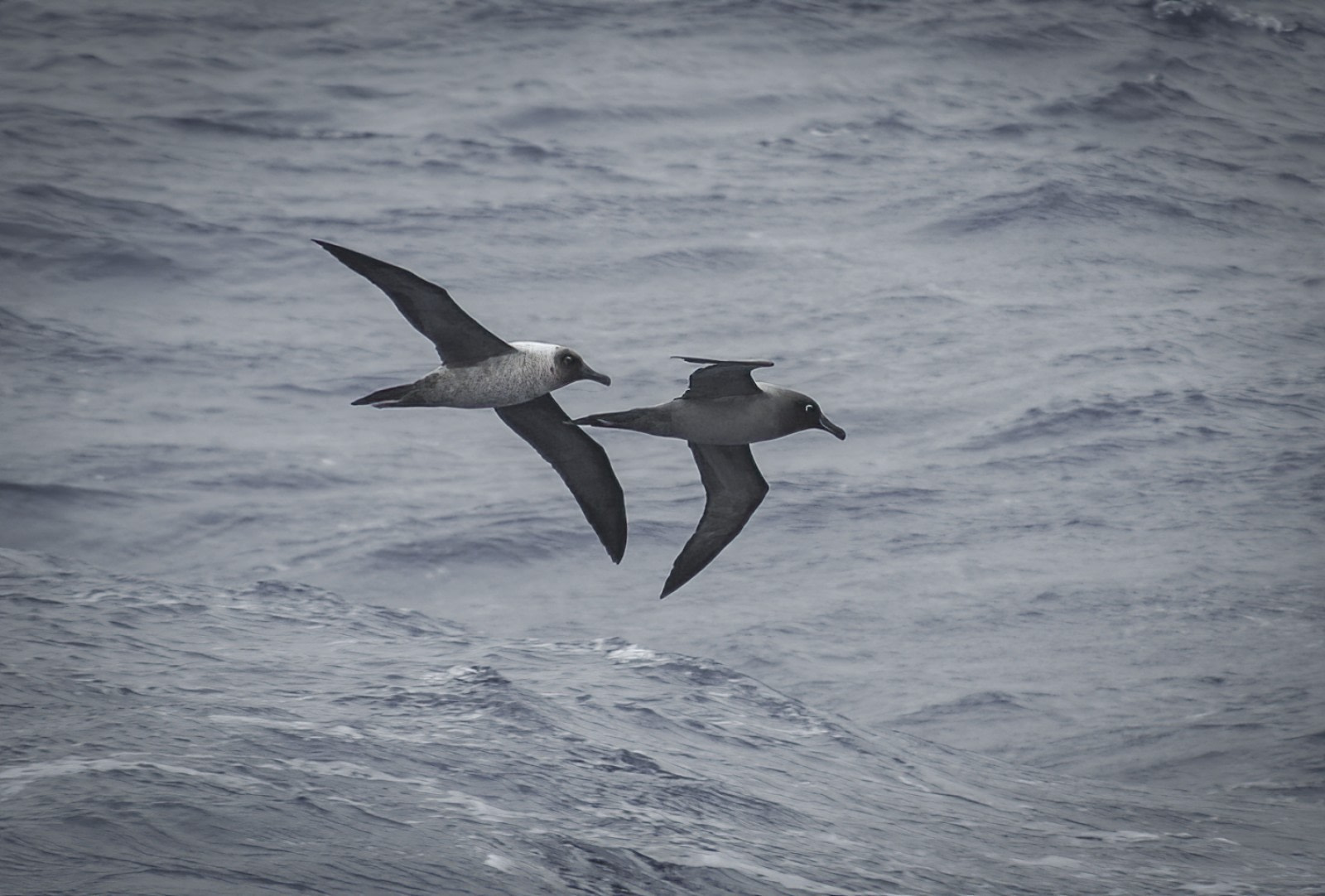This evocative image captures two seagulls soaring gracefully over a rippling, gray-hued ocean. The seagulls, positioned centrally with their wings fully extended, are heading towards the right side of the frame. The one on the left is strikingly white, with dark feathers around its eyes, a black beak, and a tail, contrasted by black-tipped wings. The seagull ahead of it is a solid charcoal gray, exhibiting a monochromatic elegance. The water below is textured with numerous small waves and ripples, a few crested with white caps, suggesting a gentle yet persistent motion. The overall scene, likely captured during the serene evening hours, is devoid of any text, focusing purely on the tranquil flight of the birds against the subtly dynamic backdrop of the ocean.